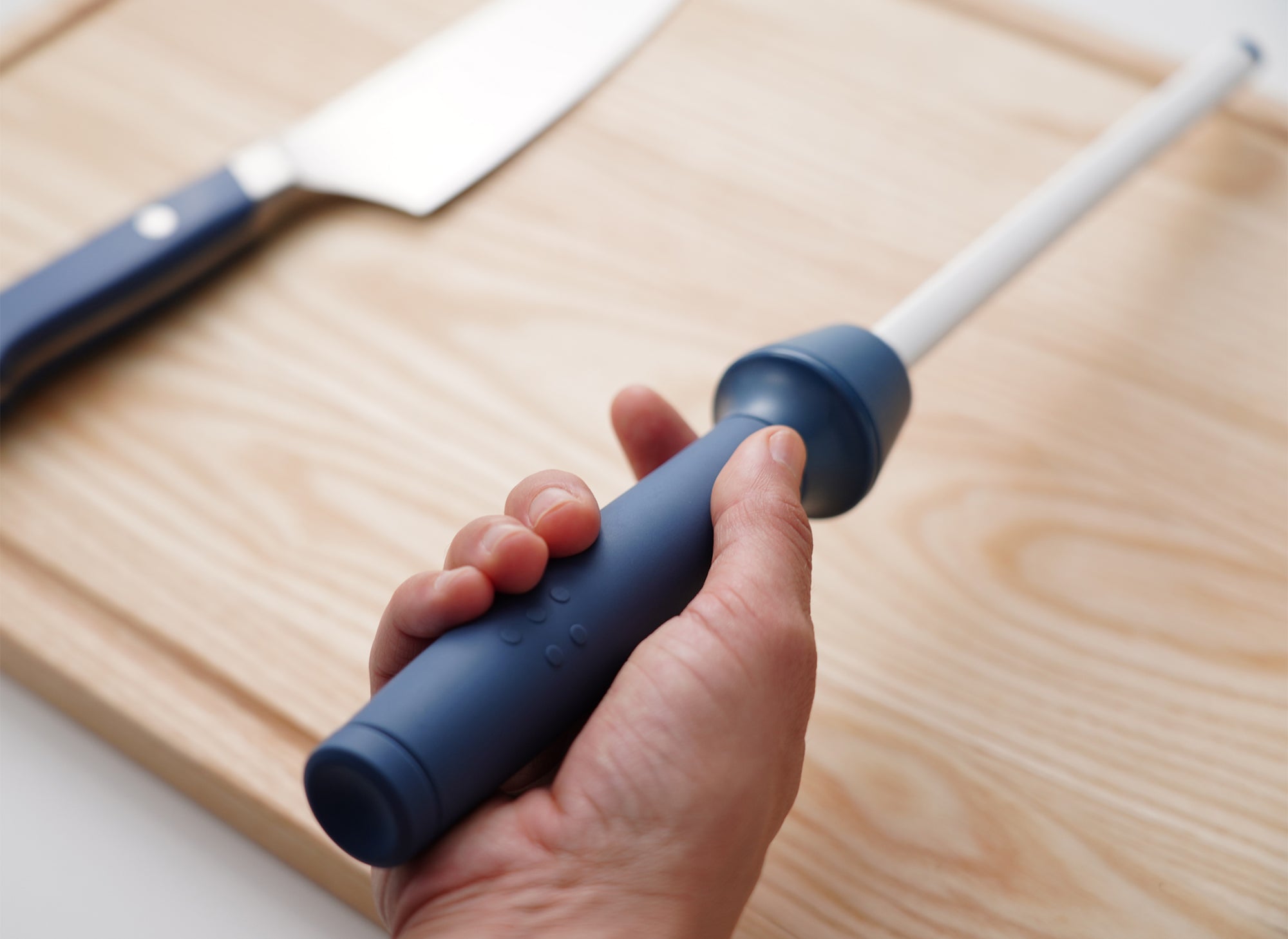In this close-up image, a male right hand is holding a knife sharpener with a distinctive blue rubber handle. The sharpener features a white, slender rod that protrudes from the handle, poised over a light wooden cutting board. To the left of the sharpener, a large chef's knife rests on the cutting board. The knife, with its blue handle and silver blade, stands out against the backdrop. The cutting board, showcasing its natural wood grain, occupies the majority of the image and sits atop a white counter, which is visible in the bottom left corner.